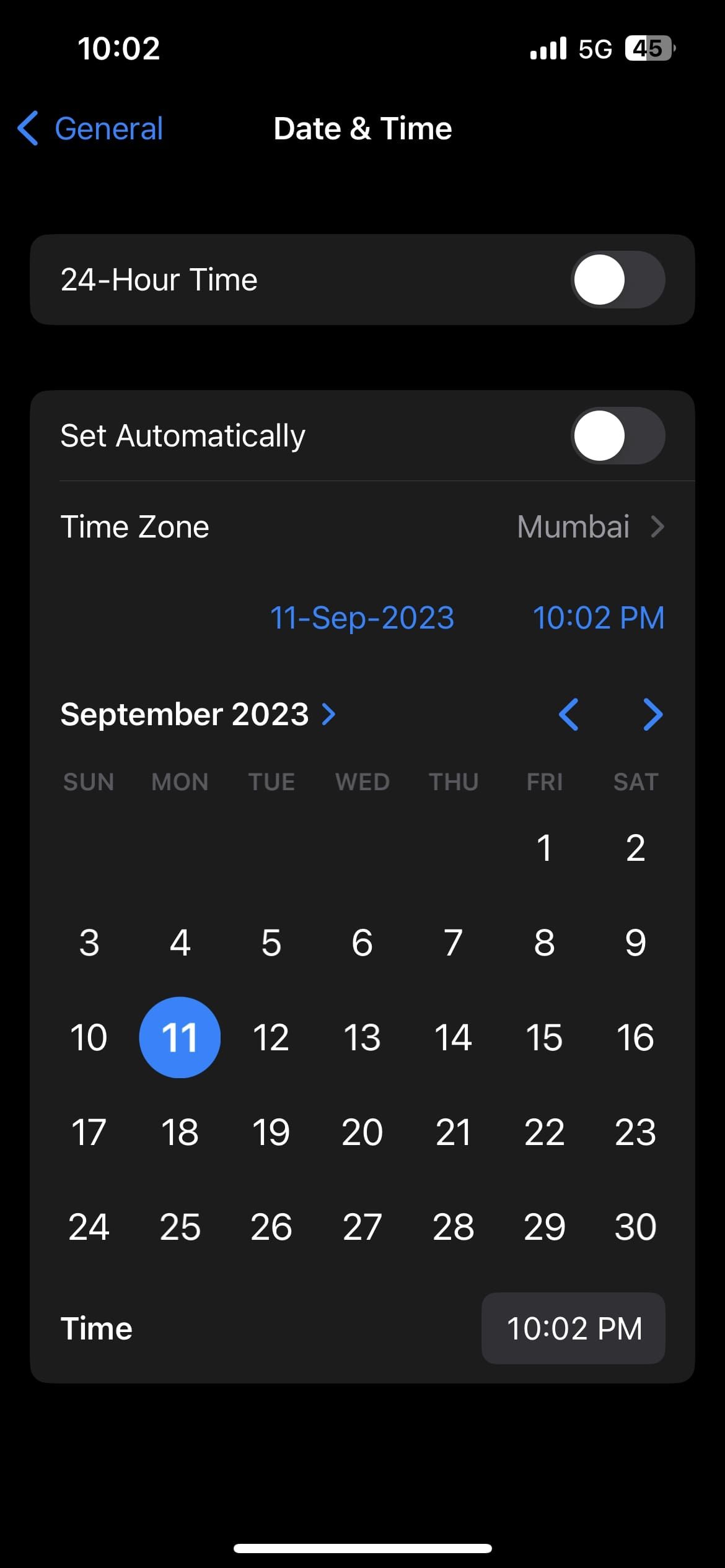The image depicts a smartphone screen displaying settings for date and time. In the top left corner, the number "1002" is visible, while the top right corner shows icons indicating a 5G cellular connection, a battery icon with "45" inside it, and other standard indicators. Below these icons, a left arrow accompanied by the word "General" in blue text is on the left. In the center of the screen, the heading "Date and Time" is prominently displayed. 

Beneath this heading, various options are listed: 

- "24-hour time": This option is currently disabled.
- "Set Automatically": This option is also disabled.
- "Time Zone": Set to "Mumbai."

Highlighted in blue font below the time zone setting is the date and time, which reads "11 September 2023, 10:02 PM."

Below this information is a calendar for the month of September 2023. The calendar layout follows the typical structure with days of the week from Sunday to Saturday at the top. The 1st of September falls on a Friday, and the calendar continues through to the 30th, which is on a Saturday. All the dates are printed in white text, but the 11th of September is distinguished by a blue circle around the date, indicating it is selected. 

Underneath the calendar, the screen displays the word "Time" on the left and "10:02 PM" on the right. The text ends here, providing a clear snapshot of the current settings for date and time on the device.